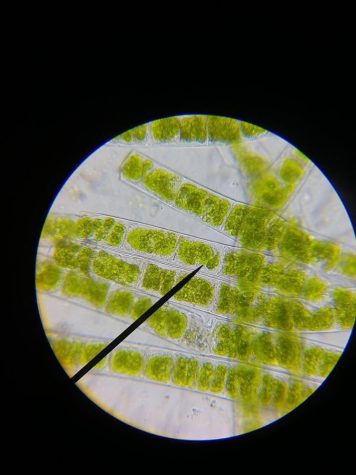This is a highly detailed close-up microscopic image. The background is entirely black, presenting a clear contrast to the white circular area in the center. Within this circular area, which appears to be the focus of the microscope, there are several long, transparent, straw-like structures filled with green content, resembling jelly-like cells or green noodles. The majority of these structures are aligned horizontally, with some overlapping and a couple standing vertically on the right side. From the 7 o’clock position on the edge of the circle, a prominent black line or arrow extends upward, pointing toward the center, similar to a pin-like structure that adds to the overall complexity of the image. The circle containing these features is nested within the larger black rectangular frame of the microscope's field of view.